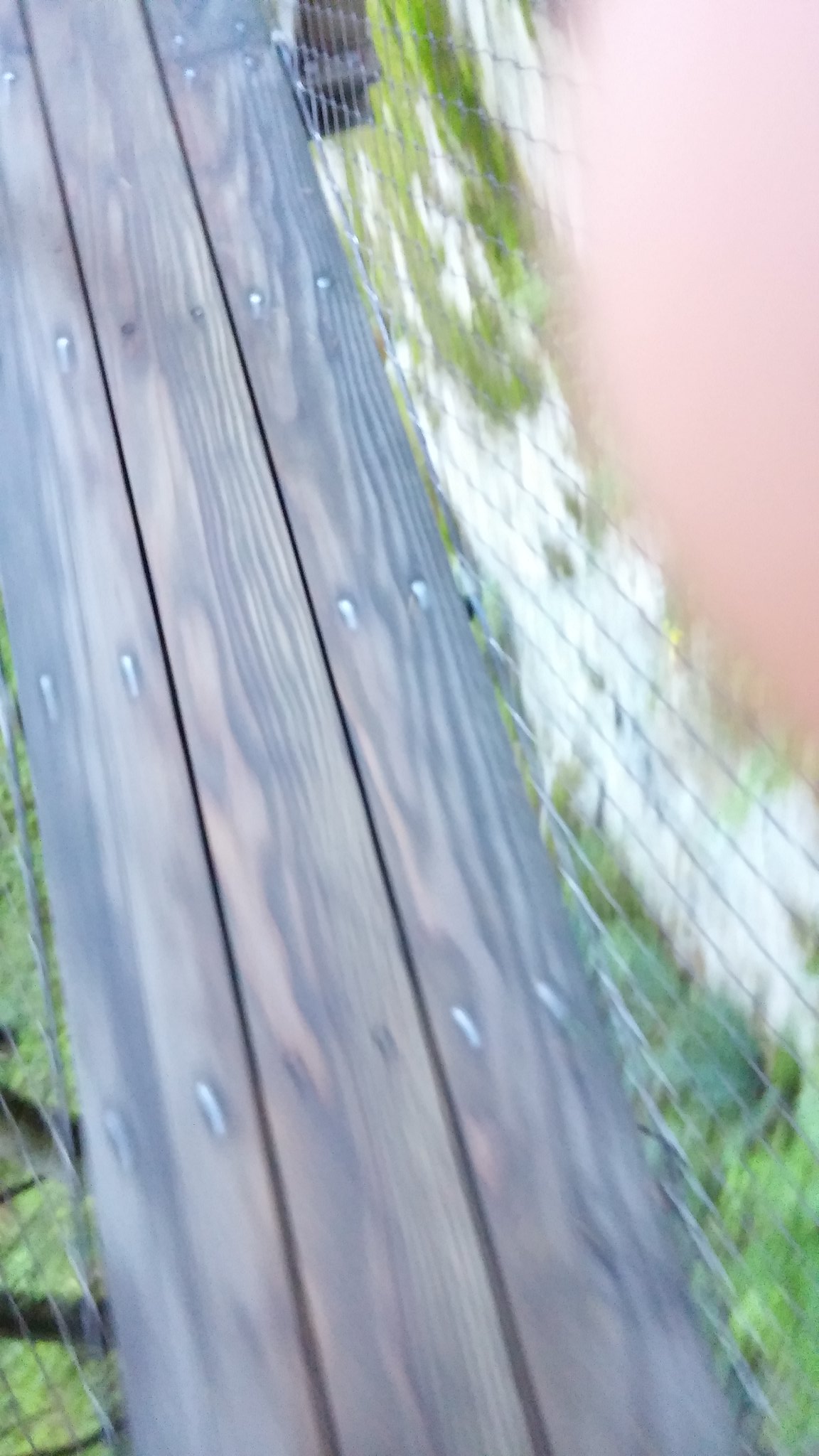A blurry, color photograph taken outdoors on a well-lit day shows three wooden planks aligned diagonally from the center bottom towards the top left of the image. These planks appear joined together with bent nails that are visible along their seams. A thumb or finger slightly obscures the top right corner of the lens, adding to the blurriness. To the right of the planks, a silver chain-link fence is noticeable, partially covered with foliage extending from the bottom halfway up the frame. There is also scattered greenery and overgrown plants, possibly with thorns and weeds, beneath and around the planks, suggesting they might have been placed as a makeshift pathway over a rough garden area. The image, in portrait orientation, has no signs of people, animals, buildings, or vehicles.